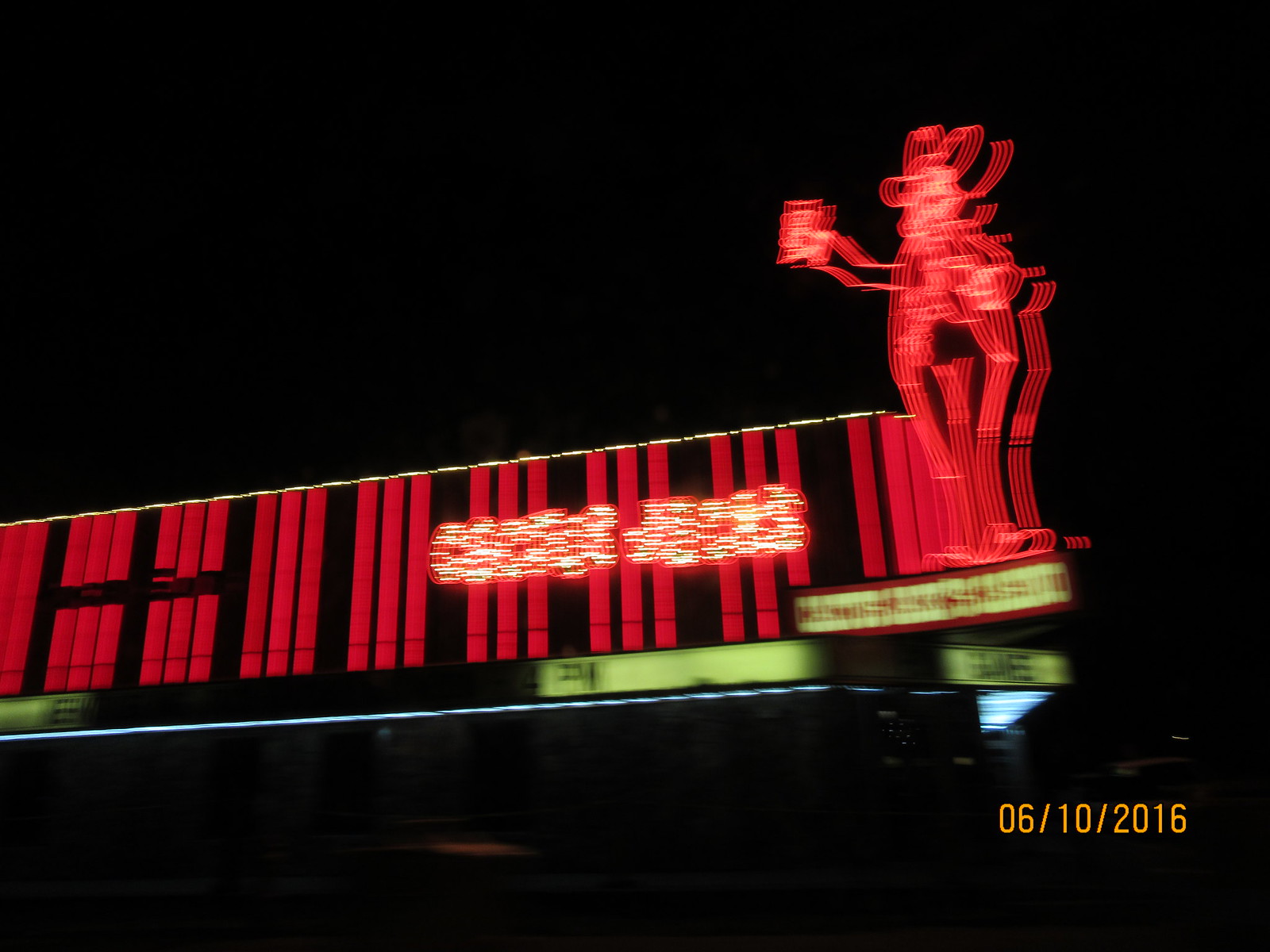Captured in motion—likely from a moving vehicle or by a person walking—this night-time photograph showcases a lively building that appears to be a restaurant or similar establishment. The image is characterized by motion blur, suggesting the photographer's movement when the shot was taken. Dominating the scene, the building is adorned with vibrant red LED lights running vertically along its structure, creating a striking contrast against the dark night sky. A prominent LED figure of a cowboy, seemingly brandishing an object, adds a touch of whimsical charm to the setting. Silhouettes of people or figures are visible around the building, contributing to the dynamic atmosphere. The photograph is date-stamped in the bottom right corner, indicating it was taken on June 10, 2016.